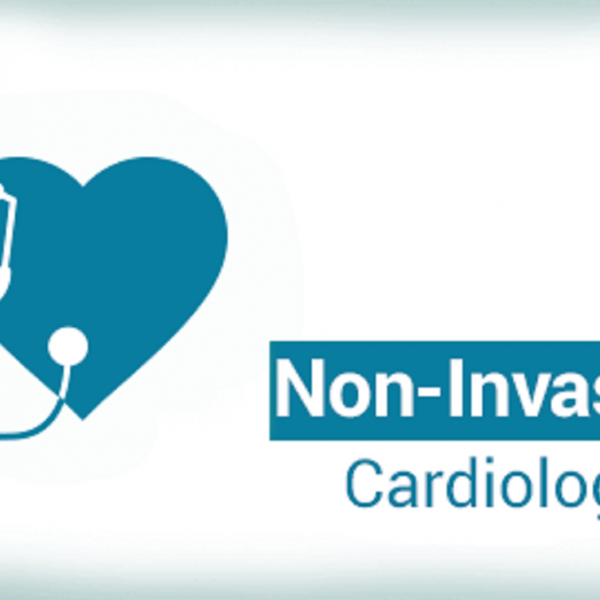The image depicts an incomplete logo on a white background with an ombre effect that transitions to grayish-blue at the top and bottom. On the left side of the image, there is a blue heart, partially cut off, with a stethoscope overlapping it. The head of the stethoscope is white, while part of its tubing is blue. To the right of the heart, white letters on a blue square spell out the partially obscured word "NON-INVASI," suggesting "NON-INVASIVE." Below this, in blue letters, is another partially cut-off word that appears to be "CARDIOLOGY." The entire image features variations of blue and white, with the details gradually fading at the edges.